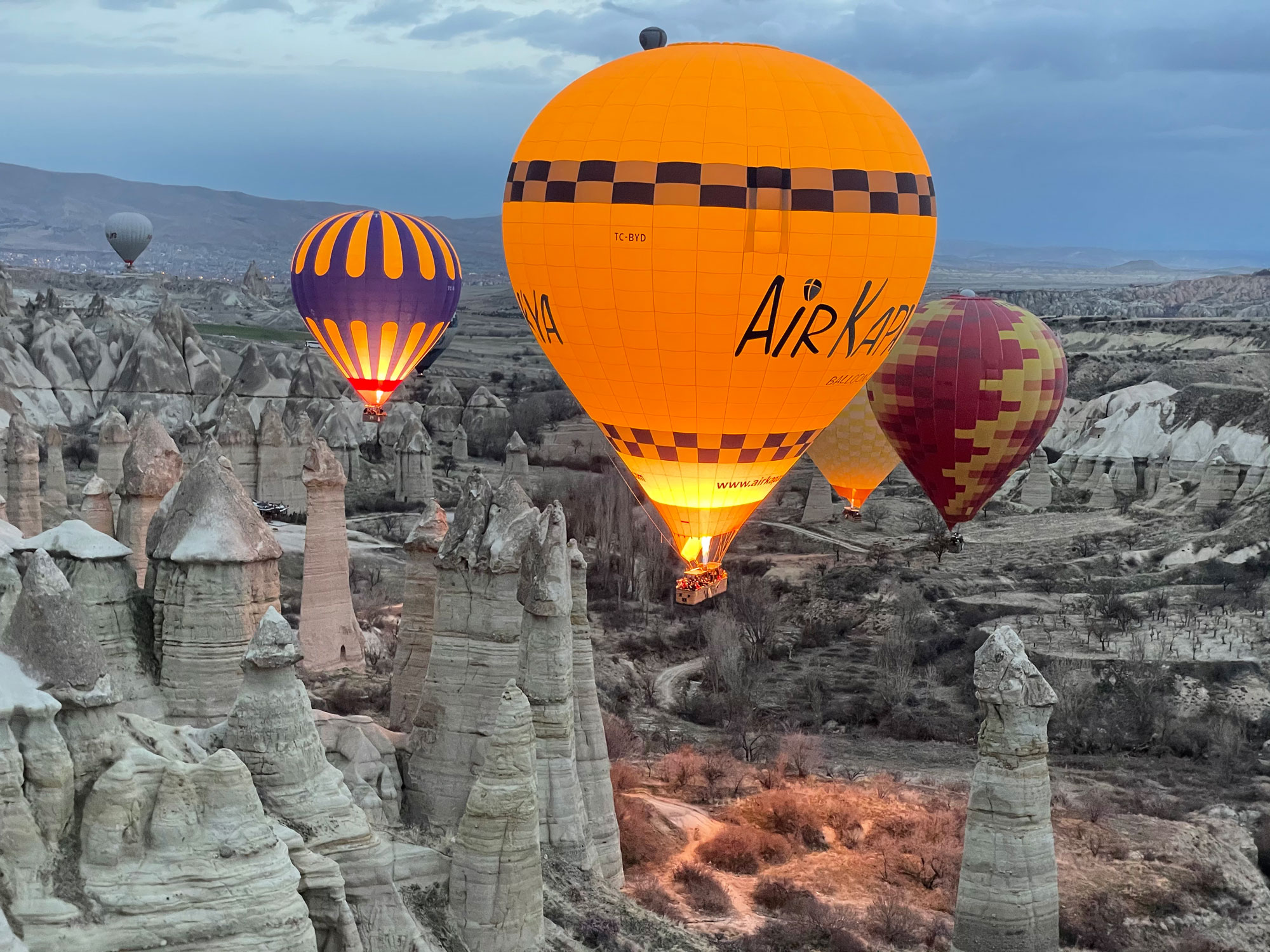In this captivating photograph, taken at high altitude, five hot air balloons are seen gracefully floating against an overcast sky. The balloons, varying in vibrant colors—orange, purple, red, blue, yellow, maroon, and gray—are similar in their classic round shape, with some adorned in intricate patterns, such as an orange balloon with a checkered blue and white band marked with “Air Carpe.” The photograph captures a moment of twilight, where the deep hues of the sunset blend with the dark clouds, casting a mystical blue tint across the scene.

The sky is filled with a thick layer of clouds, and small flames shoot up from the balloons' baskets to keep them aloft, adding a warm, flickering light to the otherwise dusky atmosphere. The landscape below features towering stone monoliths, reminiscent of ancient ruins, emerging from a desert valley covered in sandy hues and sagebrush. These formations appear as tall, pointed figures, primarily gray with light orange and red tints, adding a surreal and timeless quality to the scene. The stone structures encircle the desert-like valley, framing the dramatic flight of the hot air balloons.

In the backdrop, rugged mountains stretch across the horizon, completing this picturesque tableau. The setting, potentially a historical site with its stone formations and unique terrain, creates an enchanting and immersive visual experience, capturing the adventure and splendor of hot air ballooning over an extraordinary and ancient landscape.